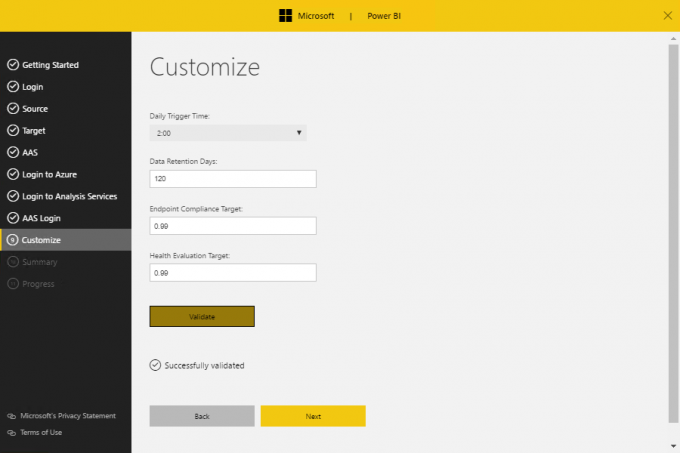The image depicts the Microsoft Power BI interface prominently positioned at the center top, featuring a yellow strip with black text. To the left, there is a vertical black strip with white or gray font displaying the following sections in sequence: "Getting Started," "Login," "Source," "Target," "AAS," "Login to Azure," "Login to Analysis Services," "AAS Login," "Customize," "Summary," and "Progress." Notably, "Customize" has a gray background, while the rest have a black background.

On the right side, the "Customize" screen is displayed, with "Customize" written in the largest font in the upper left corner. Below, there are several fields and settings: "Daily Trigger Time" set to 2 p.m. in a dropdown menu, "Data Retention Days" with a value of 120 in a white data field, "Endpoint Compliance Target" with a value of 0.99, and "Health Evaluation Target" also set to 0.99. The screen includes an orange button reading "Validate" with a black font and gray overlay, followed by a message stating "Successfully Validated." At the bottom right, there is an option to "Go Back" and an orange button.